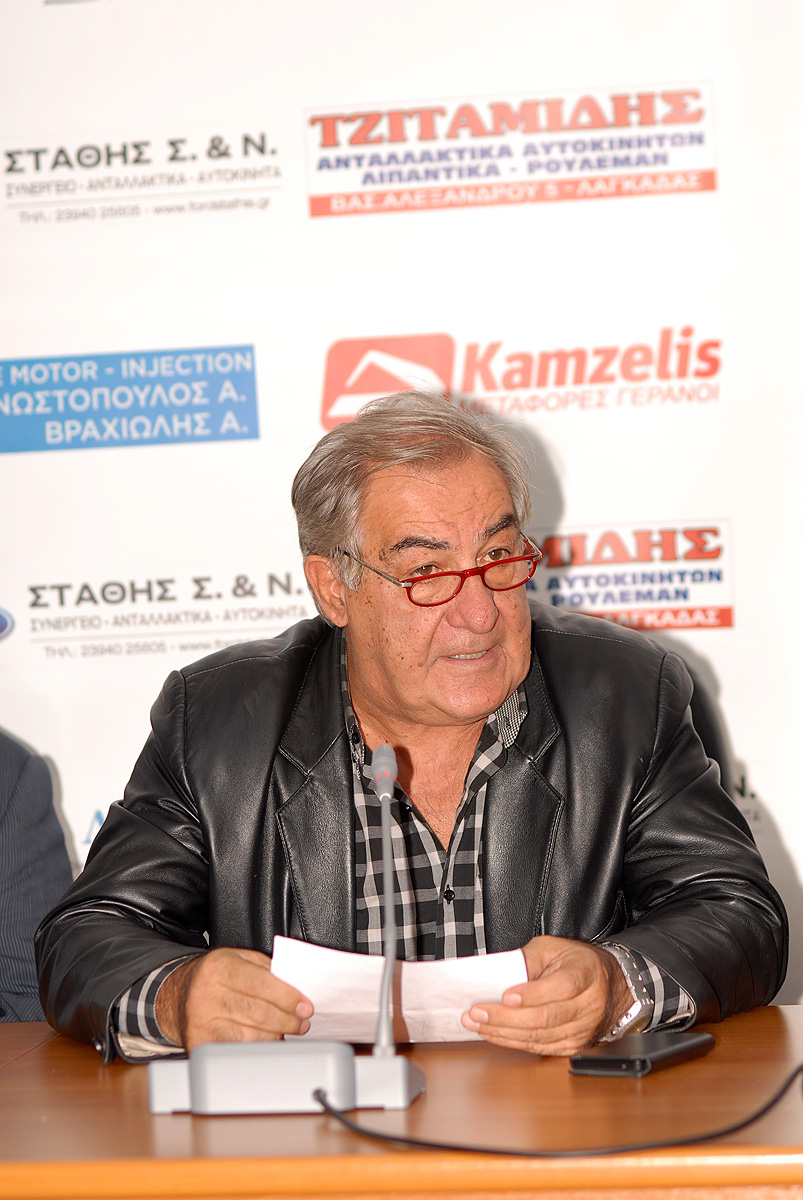In the image, an older man, appearing to be in his early 60s with graying hair, is seated behind a brown wooden table or desk. He is dressed in a black leather jacket over a black and white plaid shirt and sports distinctive red glasses. The man seems slightly heavyset and wears a silver watch on his wrist. In front of him is a microphone pointing upwards, and he holds a piece of paper in both hands, suggesting he might be addressing an audience. 

To his left, there is an object that looks like a remote control, possibly used for controlling slide presentations, rather than a smartphone. The background prominently features a white wall adorned with advertisements, possibly in Greek, with logos and names such as "TZITAMIAH," "CamXelus," and "Motor Injection." These are rendered in various colors—red and blue—and seem related to the event or conference he is attending. The man is looking off to the right, and just over his right shoulder, another individual's elbow is visible, suggesting the presence of more people at this event.